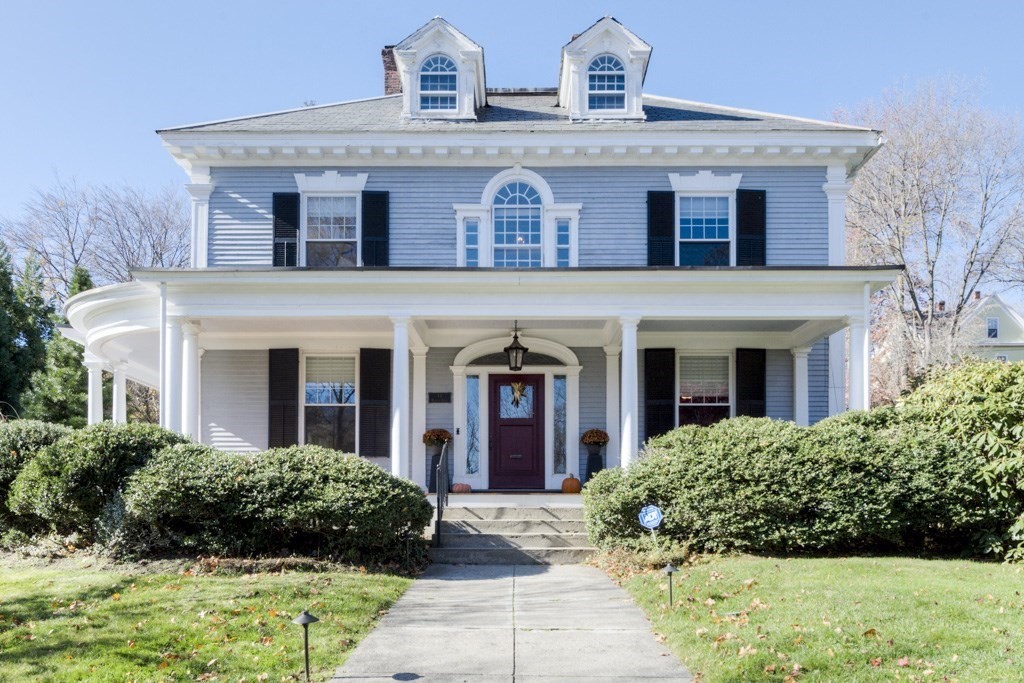This photograph showcases a well-maintained, small suburban two-story house with an attic, featuring a light blue exterior with white trim. The lush green lawn, sprinkled with brown leaves near the corners of the frame, and neatly manicured thick green bushes flank the central concrete pathway. This pathway, bordered by an ADT security sign, leads up to sturdy concrete steps and a small porch. The porch has white classical-style columns supporting white eaves, underlining a black edge of the roof above. A striking red front door with a mottled blue window, framed by vertical blue sidelights and similar columns, stands prominently beneath the eaves. Above, the house showcases blue siding with three front-facing windows: the left and right windows have white crowns and black shutters, while the central arched window boasts blue glass and column details. The gray roof features two dormer windows, each adorned with white triangular pediments, columns, and blue-arched glass. Bare brown trees surround the house, contrasting against the clear blue sky, suggesting the image was taken in a transitional season like early spring or fall. Decorative elements on the porch include a pumpkin and two flower-filled vases, adding a touch of charm to this meticulously cared-for home.